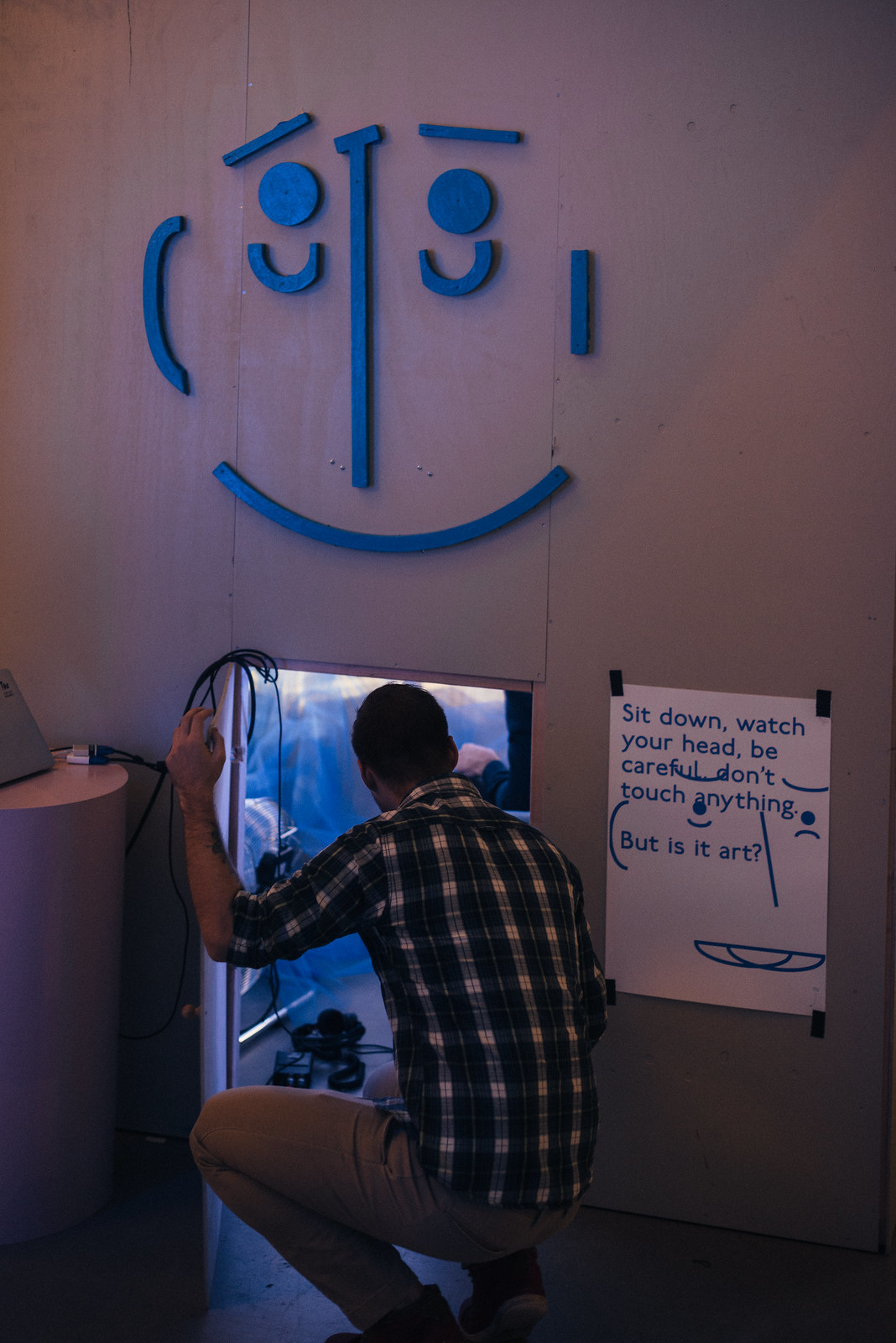The photograph, taken in portrait orientation, captures the interior of a dimly lit room with beige paneling and gray flooring. A man, appearing to be in his 30s, is the focal point of the image. He is crouched on his knees, wearing a blue and white checkered shirt with the sleeves rolled up above his elbows, tan trousers, and black trainers with gray soles. Positioned at the bottom center of the frame, he is intently examining an art installation—a plexiglass container illuminated from within, revealing a reflective silver surface and several black wires extending from the top left corner.

Directly to the man's right on the wall is a white poster, secured with black tape, bearing blue lettering that reads: "sit down, watch your head, be careful, don't touch anything, but is it art?" Above the installation is a stylized blue face made from wood, featuring geometric shapes: thin slanted rectangles resembling eyebrows, a vertical line with a slight T at the top for a nose, solid circles for eyes, U-shaped eyelids, an upturned mouth, and lines indicating ears. To the right of the man, just barely in view, is a table possibly holding a computer and more wires. The overall composition focuses on the interaction between the observer and the art piece, raising questions about the nature of art itself.